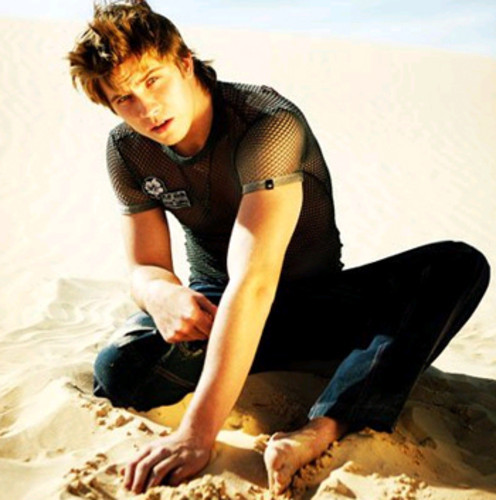The photograph captures a young Caucasian male, approximately 20-21 years old, sitting in light-colored sand at a beach, possibly at the base of a small sand dune. He has light brown, shaggy, and wet-looking hair, giving him a casually tousled appearance. The background shows a blurred strip of blue sky with faint clouds. He is barefoot and dressed in a dark, short-sleeved mesh t-shirt featuring a logo on the right chest, paired with dark denim pants. The young man is seated in a partially cross-legged position, with his left leg folded in front of him and his right leg bent. His left hand is resting in the sand, suggesting he might be digging, while his right hand is placed on his knee. He is looking directly at the camera with a slightly open mouth, adding a contemplative or questioning expression to his face.